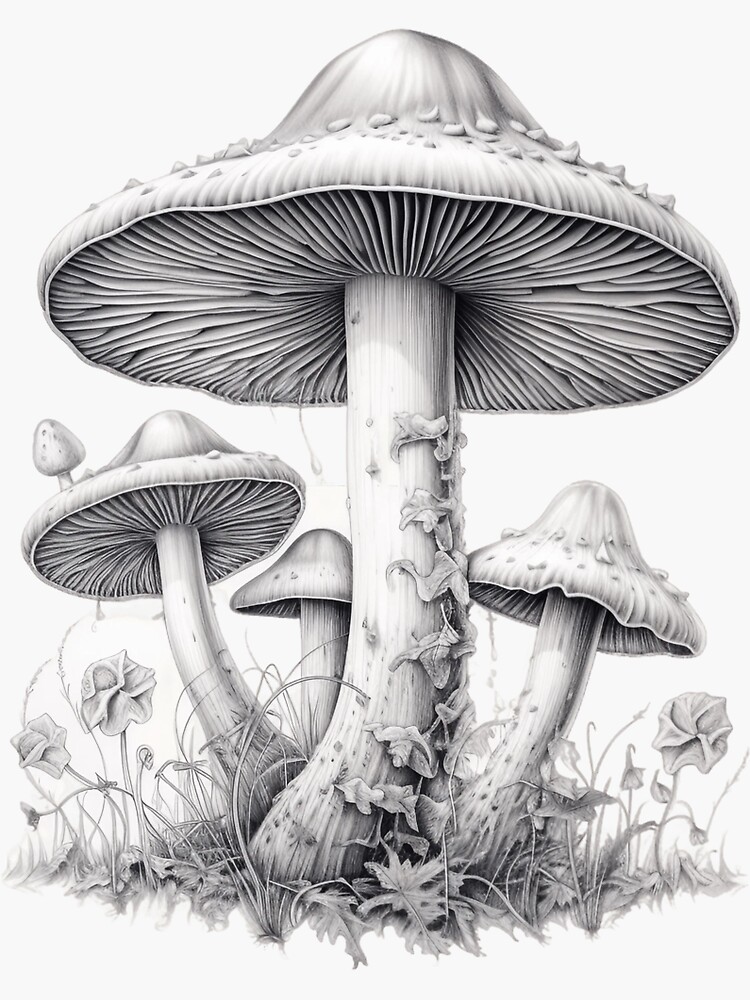This meticulously hand-drawn black and white illustration presents a cluster of mushrooms, possibly using pencil or charcoal. Dominating the center of the scene is a very large mushroom with an expansive cap that reveals intricate gill details underneath. This mushroom's long, thick stem is entwined with ivy and surrounded by leaves. Flanking the central mushroom, there are three smaller mushrooms: one to the left, slightly curved and positioned behind a taller mushroom, and another more rigid one to the right. Each of these smaller mushrooms displays various forms of undercap visibility, adding to the detailed complexity of the piece. The base of the mushrooms is interspersed with grass and small flowers, suggesting a wild, natural setting. Despite the lack of a broader background, the textured ground around the mushroom bases hints at a field-like environment.